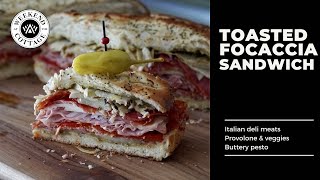The image showcases an advertisement for a toasted focaccia sandwich. Dominating the left two-thirds of this rectangular, horizontal photo, a close-up of a sumptuous, thick sandwich reveals layers of assorted cold cuts, provolone cheese, and veggies, all sandwiched between slices of Italian focaccia bread. A yellow pepper, secured with a black toothpick, adorns the top of the sandwich, while another half of the sandwich rests on a wooden cutting board in the background. On the right side, a black panel features bold white text that reads "Toasted Focaccia Sandwich," with a smaller line underneath listing "Italian Deli Meats, Provolone & Veggies, Buttery Pesto." The phrase "Weekend College" appears faintly in the top left corner, adding an intriguing touch to the image.